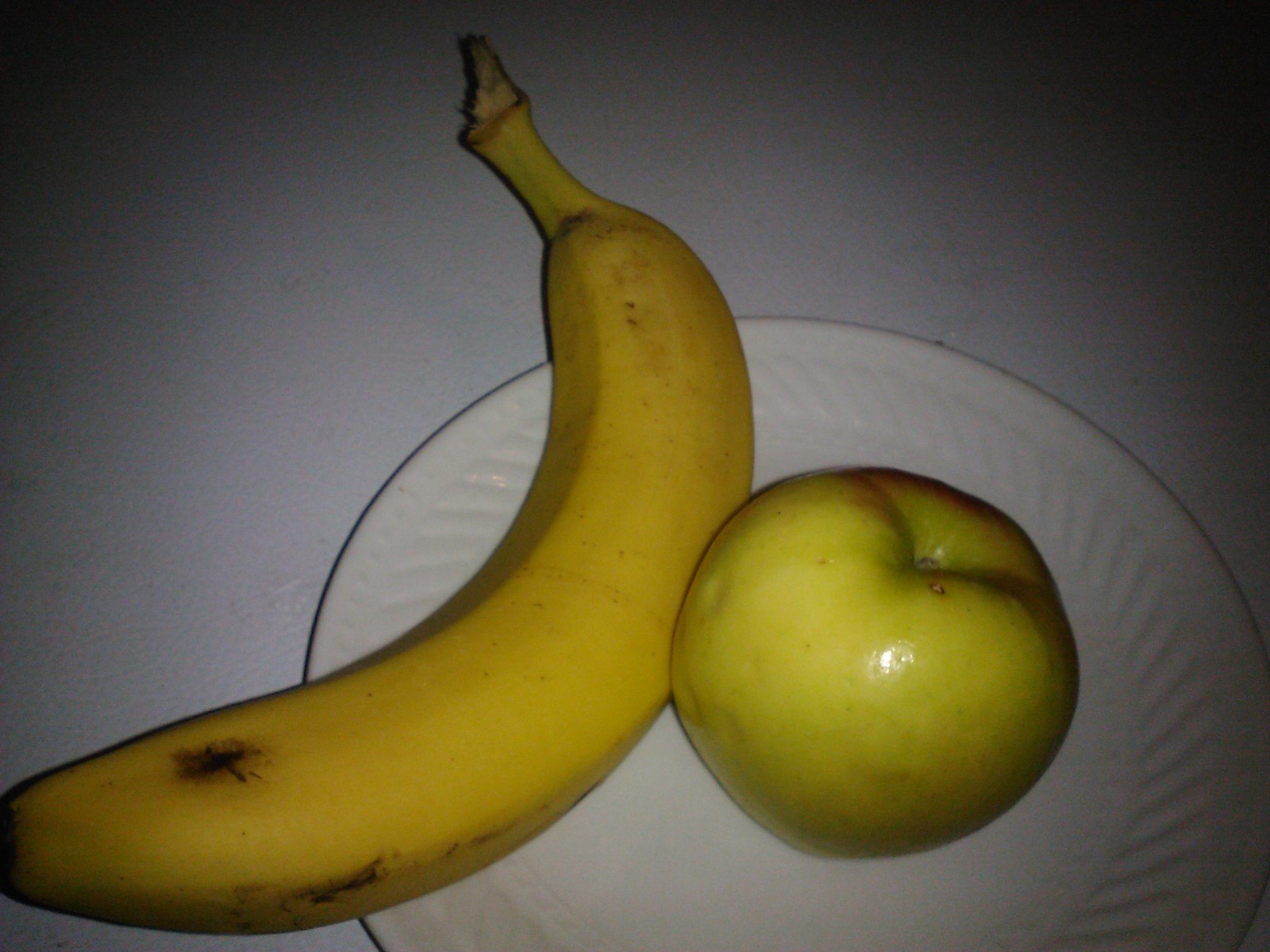In this landscape-oriented image, a vibrant tableau is set upon a gray surface. At the center sits a white plate with an ornate textured rim. On the left third of the plate, a banana extends past the plate’s edge, its skin marked with a few dark blemishes near the end while retaining its stem. Dominating the middle of the plate, a shiny apple boasts a green hue tinged with red at its apex, featuring several bruises and an evident blemish at the top. Strong focused lighting highlights the apple, casting a glossy reflection on its surface. The composition fades to black towards the top corners, adding a dramatic contrast to the scene. The bottom third of the plate is intriguingly cropped out of the frame, adding a touch of mystery to the meticulous arrangement.